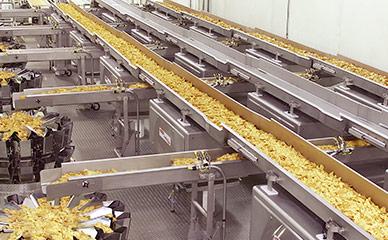The image depicts a pristine, stainless steel food processing or manufacturing plant, likely focused on producing potato-based products like french fries or potato chips. The factory floor, viewed from a second-story vantage point, is a network of metal conveyor belts and tracks that guide the golden yellow product through various stages of production. These conveyor belts span from the bottom right to the top left corner of the image, with some belts filled with the light brown, yellowish fries or chips, while a central belt remains empty. The product-laden belts lead to circular vats or barrels, positioned on the left side of the image, where the fries are either being cooked or prepared further. The entire facility appears clean, sterile, and entirely automated with no visible personnel, emphasizing its mechanical nature.